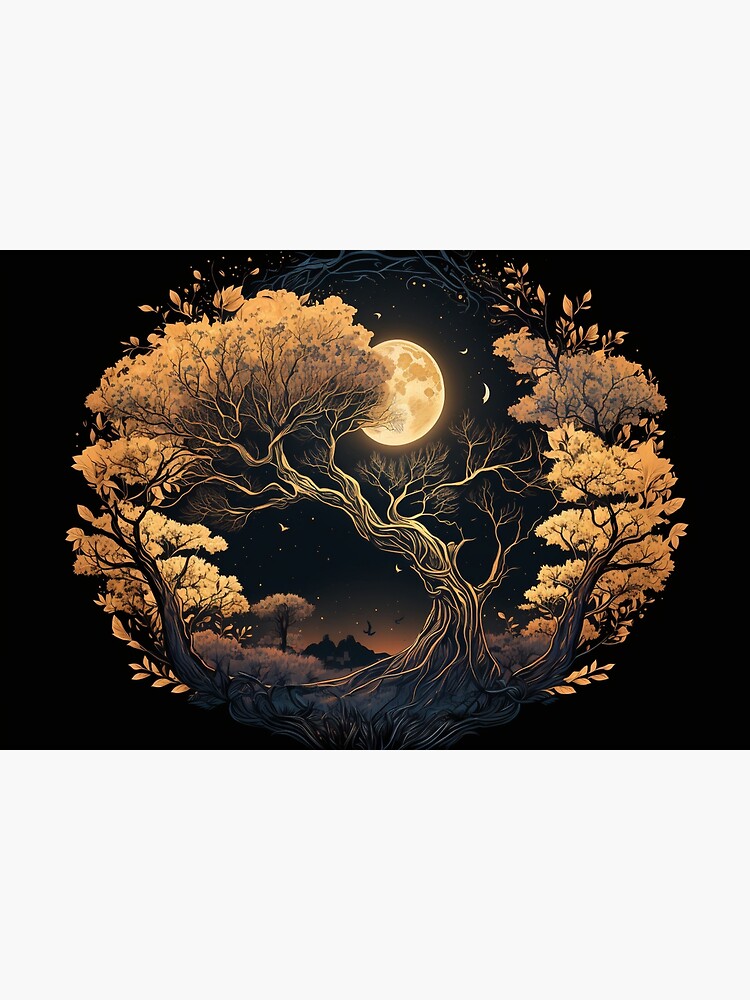This artwork illustrates a dramatic night-time scene set in an outdoor fall setting, dominated by a glowing orange and golden palette. Central to the composition is a large, slightly bent tree whose leaves billow to the left. The tree stands within an oval-shaped arrangement of other trees, their branches extending wildly and forming a circular pattern that defines the artwork's borders. The background is a deep black, emphasizing the night-time ambiance.

Encompassed within this oval are three interconnected trees rooted at the bottom of the image, with one central tree arching towards the upper left, flanked by trees on either side stretching up along the circle's borders. Behind this arboreal display, a bright, glowing yellow full moon shines prominently, partially obscured by the orange foliage. The sky features a sprinkle of stars and flying black birds, with distant hills and a grassy area adding depth to the scene.

The color scheme is predominantly dark with intense autumnal hues, creating a vibrant contrast against the night sky, evoking a sense of drama and dynamic movement through the curvy, wild tree branches and varying shades of orange leaves.